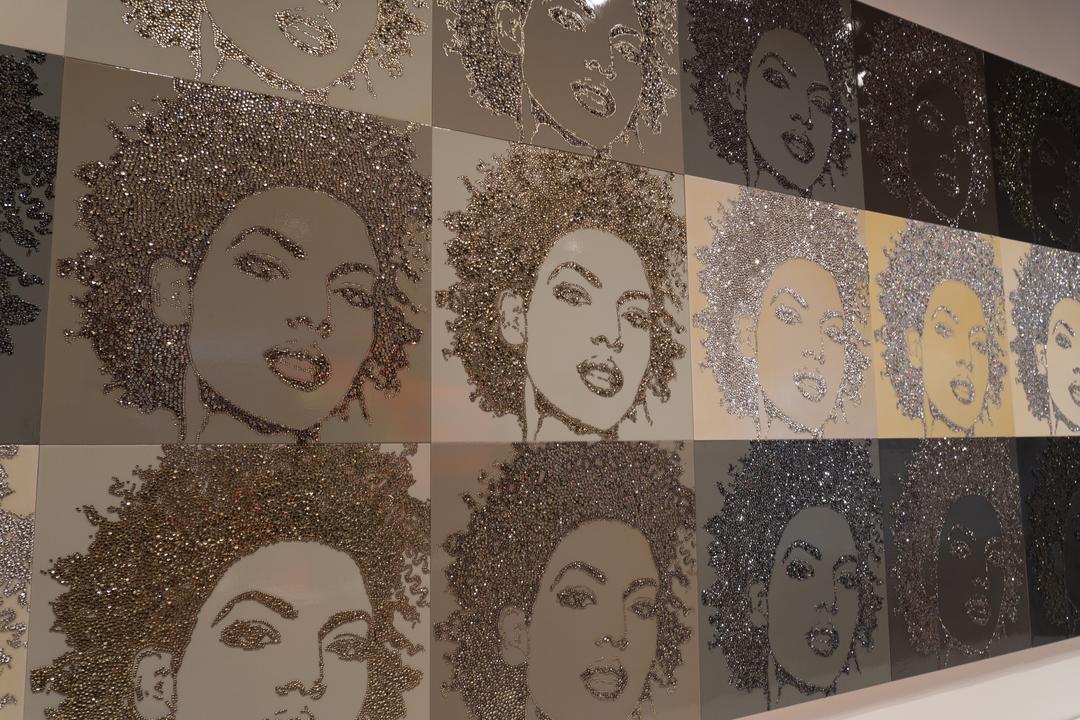The image depicts an art installation inside a modern museum or exhibit, featuring a striking wall of artwork. The artwork is composed of three rows of square tiles, each showcasing a portrait of an African-American woman's face. This face, reminiscent of the Lauryn Hill album cover art, is rendered using different shades of glitter and sparkling materials that range from very light to very dark. The glitter varies in color across the tiles, contributing to the intricate shading of the woman's face and hair. Each individual tile offers a unique background color, incorporating hues from beige or yellowish-white to deep black, creating an engaging visual gradient. The juxtaposition of these tiles forms a cohesive yet varied large-scale image that captivates viewers with its detailed craftsmanship and shimmering beauty.